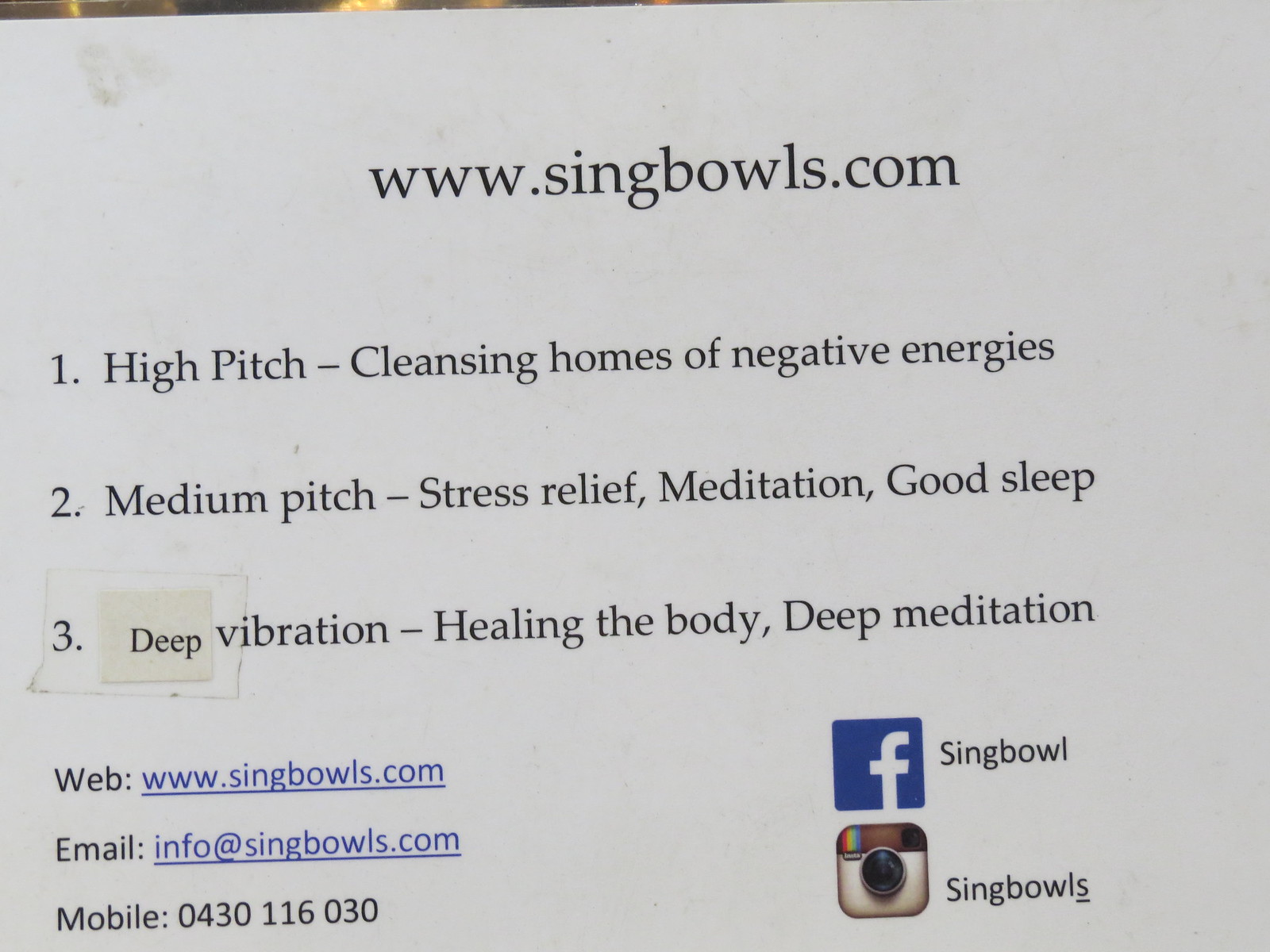The image appears to be a photograph of a printed sign or a page from a book showcasing information about singing bowls, specifically from www.singbowls.com. The page, which is predominantly white, features both black and blue fonts and various icons. At the top, it prominently displays the website address: www.singbowls.com. The content following this includes a detailed list describing the benefits and uses of different pitches of singing bowls:
1. High-pitch for cleansing homes of negative energies.
2. Medium pitch for stress relief, meditation, and promoting good sleep.
3. Deep vibration for healing the body and facilitating deep meditation.

Interestingly, the word "deep" appears to be a cut-out piece of paper that has been taped over something else, suggesting a possible correction or emphasis.

Further contact information is listed, including an email address (info@singbowls.com) and a mobile number (0430116030). The bottom right corner of the page features social media icons: a Facebook icon labeled "singbowl" and an old-timey Instagram icon labeled "singbowls," with the 'S' underlined.